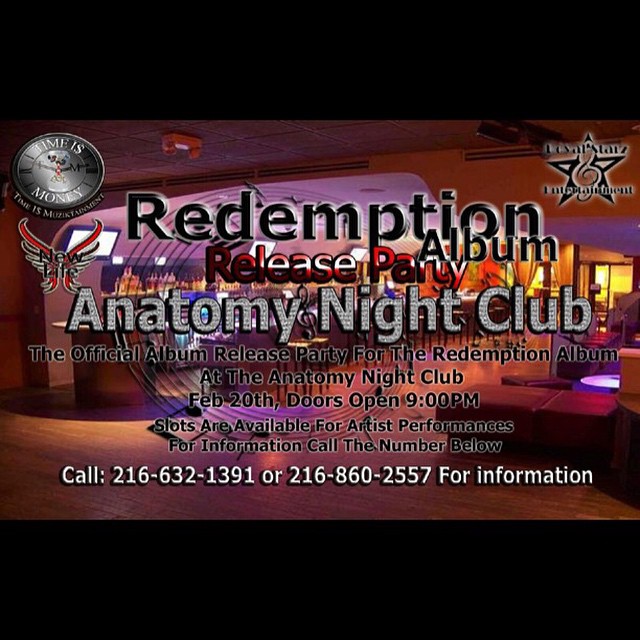The image is a flyer for an official album release party at a nightclub called Anatomy Nightclub. The background features a dimly lit, empty nightclub with ambient lighting, showing a bar with stools, a variety of liquor bottles, and a mounted TV. To the right, there's a lounge area with seating. Black bars frame the top and bottom of the flyer, giving it a distinct ad-like appearance. 

At the top left corner, there is a logo that reads "Time is Money. Time is Music Tainment." The prominent header in the middle of the flyer announces in large text, "Redemption Album Release Party." Below that, in various text formats, it states, "Official album release party for the Redemption album at Anatomy Nightclub, February 20th, doors open at 9 p.m." The flyer also mentions that slots are available for artist performances and provides additional contact information, instructing viewers to call 216-632-1391 or 216-860-2557 for more details.